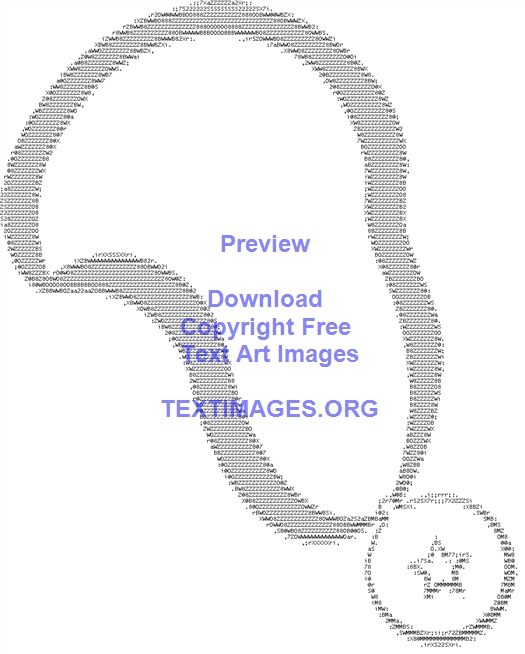This image depicts an intricate piece of ASCII art portraying a medal of achievement designed entirely with keyboard characters. The artwork features a circular medallion adorned with the outline of a star at its center. The medal hangs from a textured gray ribbon, meticulously crafted to appear as though it would be worn around someone's neck. The overall graphic is set against a plain white background.

In the center of the image, purple text prominently reads, "Preview," followed by "Download Copyright-Free Text Art Images" beneath it. At the bottom of the image, the website "TextImages.org" is displayed in uppercase letters, also in purple. The ASCII art comprises a range of characters, including Z's, R's, 8's, and dots, contributing to the detailed formation of both the ribbon and the medallion.